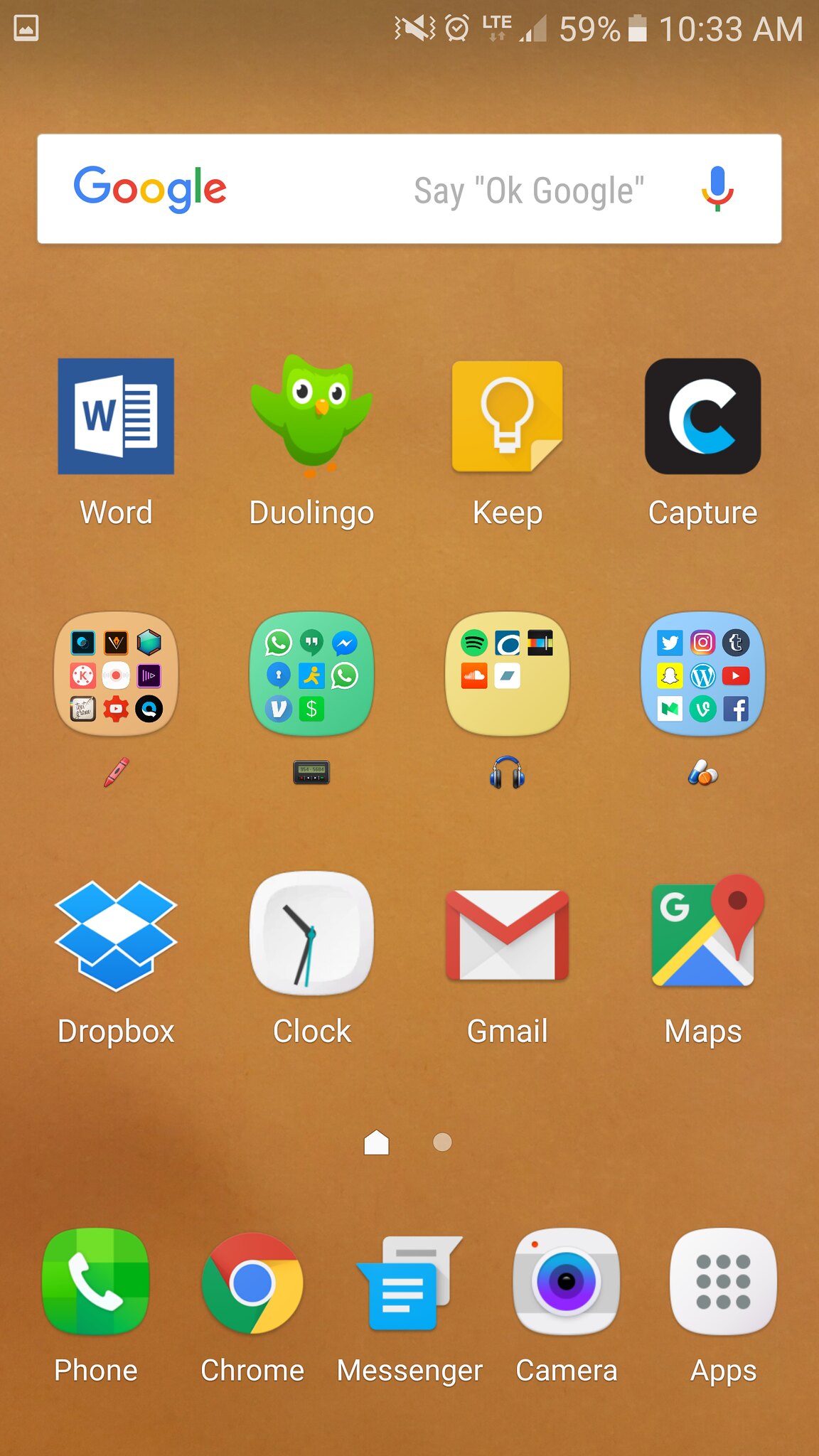This image is a screenshot of a home screen on either an Android or Samsung device. At the top, there is a white bar featuring the Google logo and the text prompt "Say OK Google," accompanied by a microphone icon on the right. Beneath this bar, the visible apps include Word, Duolingo, Keep, and Capture.

In the central section, there are four folders. The first folder icon depicts a red crayon, the second one features a communication device emoji, the third folder displays a headphone emoji, and the fourth one shows two pill emojis.

On the third row, the apps visible are Dropbox, Clock, Gmail, and Maps. At the bottom of the screen are the prioritized apps for easy access, which include Phone, Chrome, Messenger, Camera, and the button to access all apps.

The background of the home screen is a plain brown color. The status bar indicates the phone is at 59% battery and the time the screenshot was taken is 10:33 a.m. The device has two bars of signal strength and is connected to an LTE network.